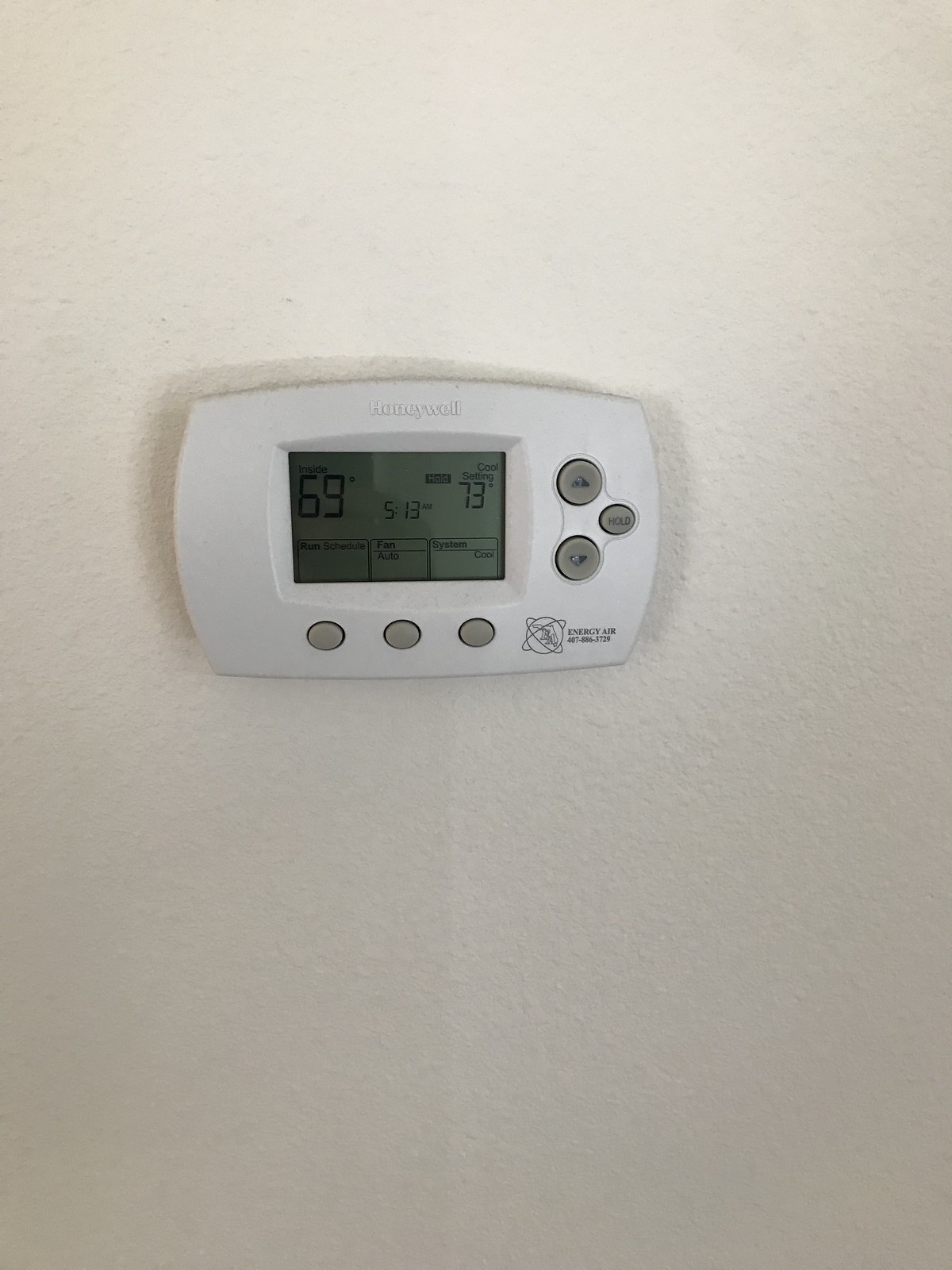This is a detailed color photograph of a Honeywell home thermostat mounted on a white textured wall. The thermostat features an electronic display screen prominently positioned in the center. To the right of the screen, there are three control buttons arranged vertically, which resemble arrow keys. Just below these arrow buttons is a smaller, oval-shaped button labeled "Hold." Beneath the display screen, there are three additional small buttons without any visible text indicating their functions.

On the display screen, the thermostat is set to 69 degrees Fahrenheit. Flanking this temperature on the right side is the current desired temperature setting. The current time, displayed in the center between the two temperature readings, is 5:13. Additionally, there are several other small icons and boxes representing various functions and control settings.

The brand logo, Honeywell, is visible along with a distinctive energy-saving feature logo that resembles an Earth orbited by Saturn-like rings. This image captures the detailed layout and functionality of a contemporary Honeywell thermostat designed for home climate control.